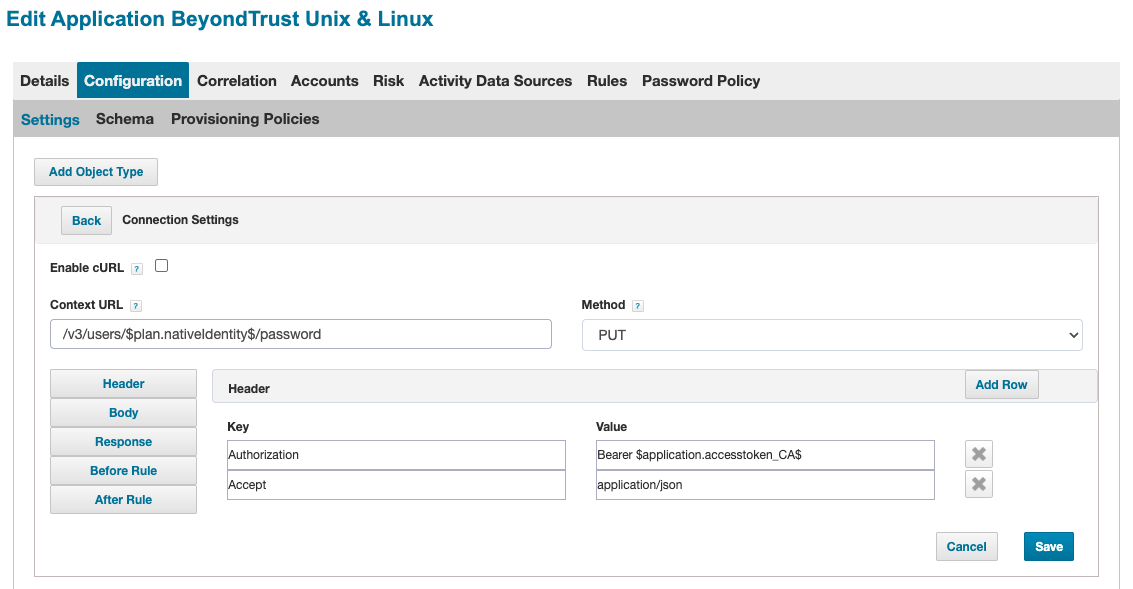On the displayed settings page for the "Beyond Trust Unix and Linux" application, various navigation tabs appear prominently at the top. These include "Details," "Configuration," which is currently highlighted in blue, "Correlation," "Accounts," "Risk," "Activity Data Sources," "Rules," and "Password Policy." Below these primary categories, sub-categories labeled "Settings" (also in blue), "Schema," and "Provisioning Policies" are present.

Two prominent buttons labeled "Add Object Type" and "Back" are positioned near a section titled "Connect Settings." This section consists of two checkboxes: "Enable CURL" and "Context URL," both of which appear next to an accompanying link.

Further down, under the "Method" category, the chosen method is "PUT." Accompanying this are headers defined as "Key" and "Authorization," with a relevant "Value" specified as "Bearer Application Access Token CA$, Application JSON." The content predominantly appears against a simple white background, highlighted only by the technical specifics such as "Response Before Rule" and "After Rule." The Context URL concludes with the version string "v3.0.0.0.0.0.0.0.0."